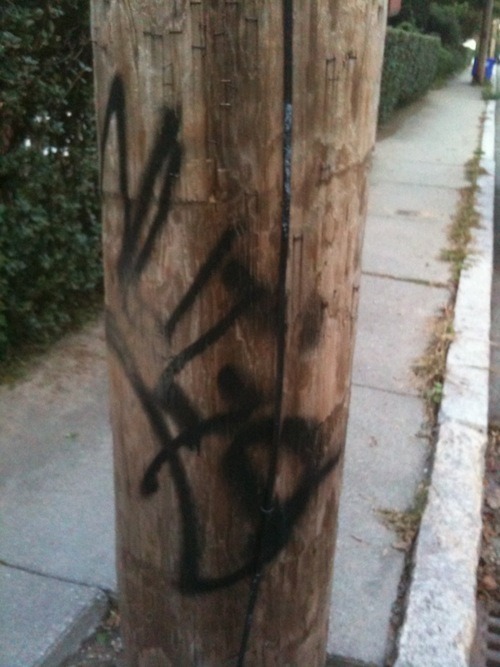The image features an up-close view of a medium to dark brown wooden light pole with black graffiti sprayed on it, reading "M-I-T-G." The photograph, seemingly taken outdoors, captures only the lower part of the pole, cutting diagonally from the top left to the bottom right of the frame. The image is somewhat blurry and appears grimy, suggesting something might be on the lens. Behind the pole, there is a concrete sidewalk stretching from the bottom to the top of the frame. The sidewalk is flanked by overgrown plants and cracks with grass on the right side, bordered by a concrete edge. To the left, a well-maintained hedge of green leaves runs diagonally from mid-page to the top right corner. In the distant background, a blue recycling bin is faintly visible.